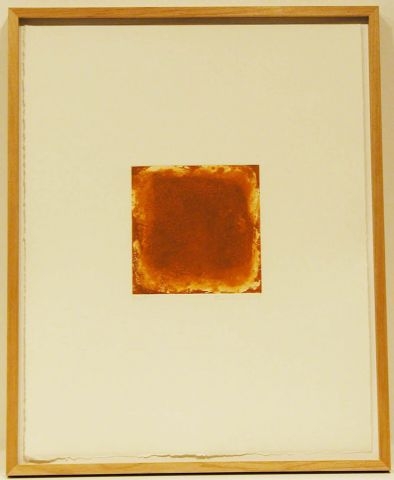This vertically-oriented image captures a framed piece of artwork set against a largely cropped-out beige wall. The frame itself is a thin, medium-brown wood that elegantly borders an ivory matte background. At the center of this matte lies a small, colorful square piece of art. The artwork showcases a rough, textured square with a reddish-brown or golden-brown center encircled by yellow hues resembling flames. Although the central image lacks a defined form, its layers and juxtaposition of brown and yellow create a striking, if abstract, visual effect. Notably, the bottom edge of the matte shows some roughness, as if slightly torn. This composition highlights the contrast between the minimalist frame and the vivid, fiery artwork within.